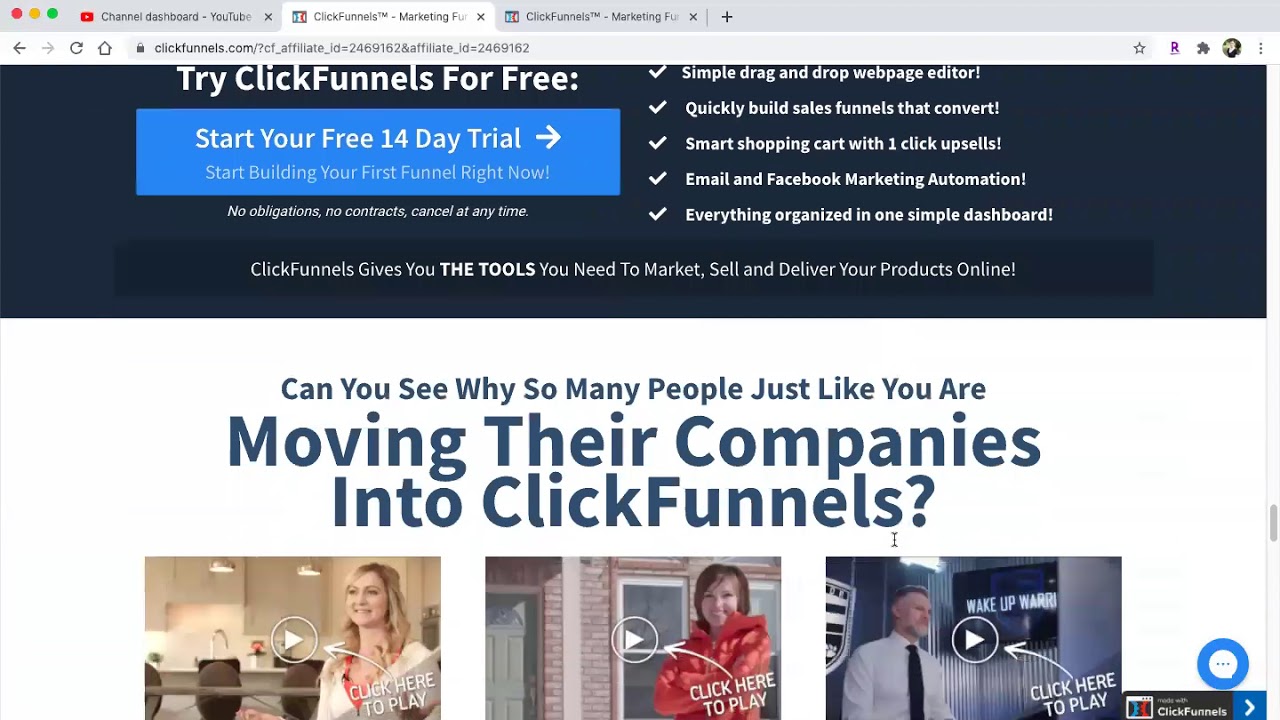**Screenshot of ClickFunnels Website on Macintosh Laptop**

The image is a screenshot captured from a Macintosh laptop, identifiable by the dark grey bezel at the top. The bezel features the standard red, orange, and green circles commonly associated with the Safari browser.

At the top right, there are browser tabs. The unselected tab features a YouTube icon (a rectangular logo with a white triangle) accompanied by the text "Channel Dashboard - YouTube," partially cut off and with an 'X' to close it. The selected tab is white and shows an icon with teal and red bent lines, titled "ClickFunnels™ - Marketing FUR..." and an 'X' for closing it. To its right is an identical, unselected tab in grey.

Below the tabs is the browser navigation bar. It contains dark grey back and forward arrows (the forward arrow is greyed out, indicating it is not clickable), a refresh button, and a home button. The URL bar includes a secure lock icon followed by text: "ClickFunnels.com/7cf_affiliate_id=2469162." Adjacent to the URL bar, a dark blue bezel displays a bold white call to action "Try ClickFunnels for free."

On the main webpage, a mid-blue button reads "Start Your Free 14 Day Trial," with an accompanying right-pointing arrow. Below this, in light blue text, it states, "Start building your first funnel right now!"

On the right side, there are several bullet points in bold white text, each preceded by a bold white check mark:

- Simple drag-and-drop website editor!
- Quickly build sales funnels that convert!
- Smart shopping cart with one-click sales!
- Email and Facebook marketing automation!
- Everything organized in one simple dashboard!

Underneath, in grey italics, there is a message: "No obligations, no contracts, cancel at any time."

Centrally, the page reads: "ClickFunnels gives you the tools you need to market, sell, and deliver your products online." In bold blue text, it continues, "Can you see why so many people just like you are," followed by large bold text, "moving their companies into ClickFunnels."

Several testimonial images are featured:

1. **Woman in White Shirt**: A smiling blonde woman wearing a white shirt with an orange undershirt, set against a cream-colored background adorned with cascading silver lights. A play button overlay is visible.

2. **Woman Next to Brick Building**: A woman with short brown hair in an orange jacket, standing beside a red and brown brick building with windows and a glass door, captioned "Click here to play" with a play button.

3. **Man in White Dress Shirt**: A man in a white shirt and black tie against a multicolored background with silver and white elements, labeled "Click here to play" with a play button.